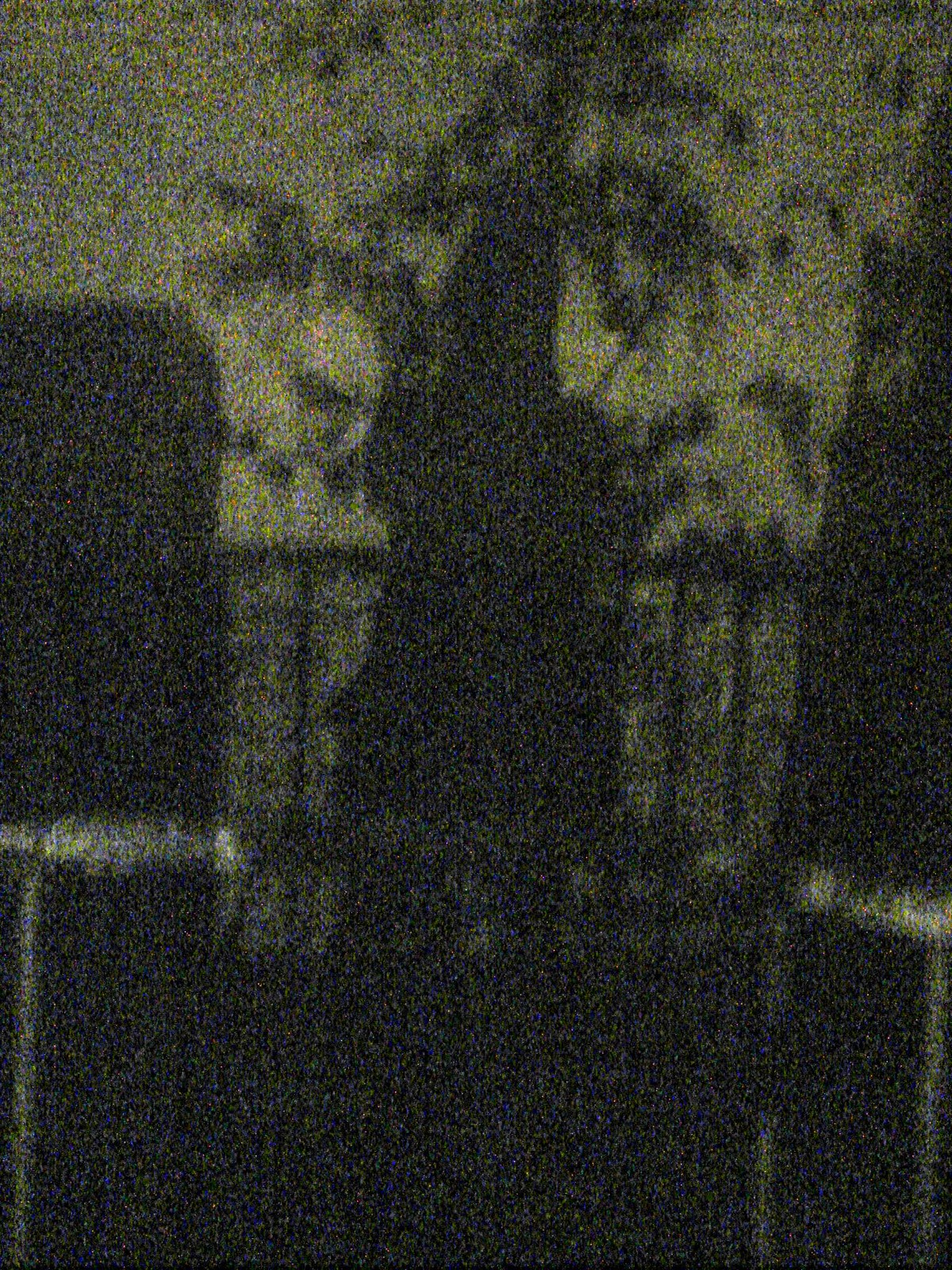The image is a dark and grainy black-and-gray scale photograph, featuring obscure, shadowy outlines and indistinct silhouettes. At the center of the frame, there is a slightly tall structure resembling the outline of a tree with a thick, stout trunk. The tree's upper portion is adorned with sparse branches and leaves, contributing to its skeletal appearance. On either side of the tree, there are column-like structures of a shorter height, flanking the main focal point. A fence with vertical bars, which reaches halfway up the tree's trunk, spans the foreground, adding to the scene's somber and enigmatic atmosphere.